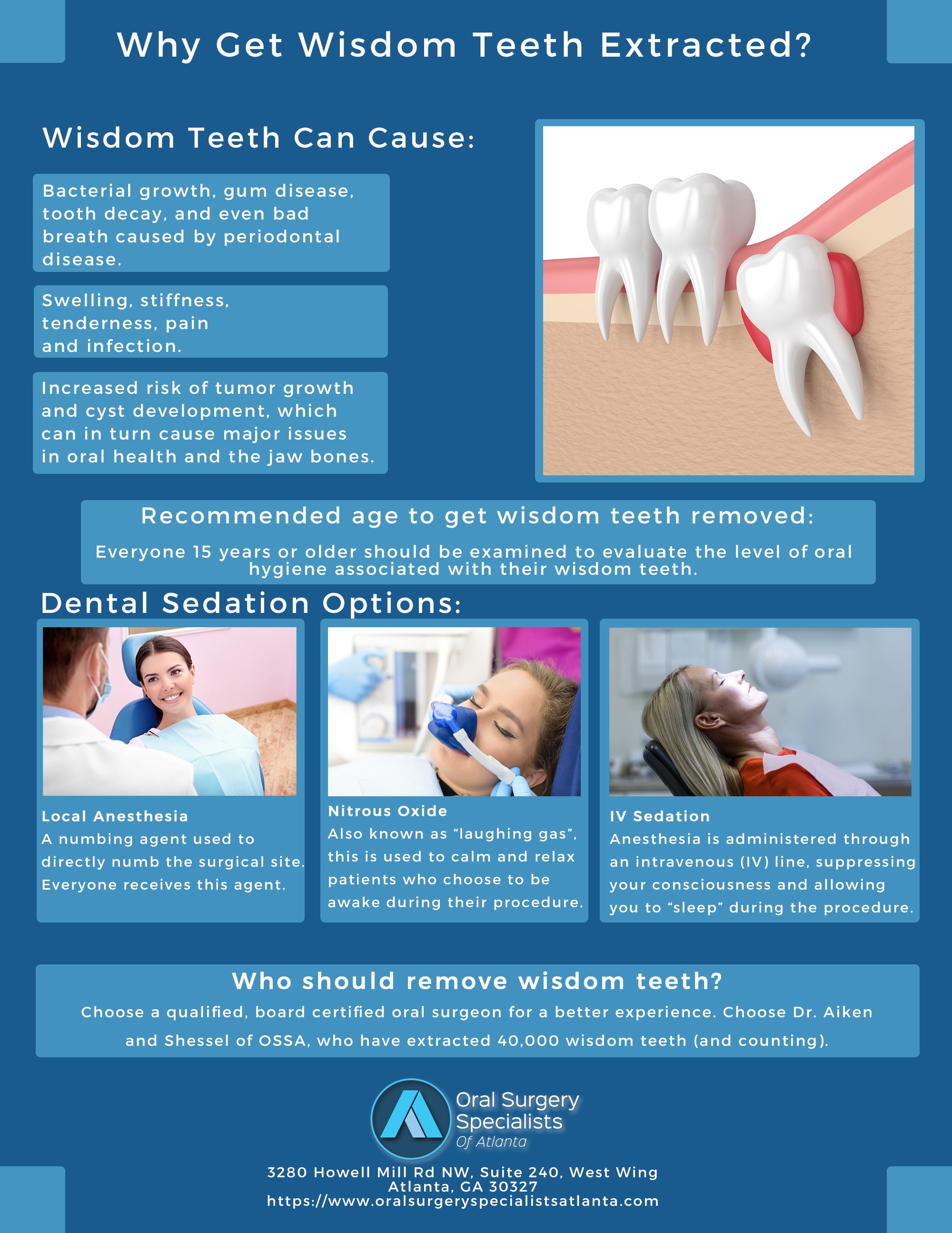This image features a detailed advertisement for the Oral Surgery Specialists of Atlanta. The advertisement has a predominantly blue background with several images and detailed text. The central theme emphasizes the importance of getting wisdom teeth extracted. The text explains that wisdom teeth can lead to numerous oral health issues, including bacterial growth, gum disease, tooth decay, periodontal disease, swelling, stiffness, tenderness, pain, infection, and even increased risks of tumor growth and cyst development, all of which can significantly impact oral health and jaw bones.

Accompanying the text are various visual aids: a 3D illustration of a wisdom tooth, a series of photographs that depict patients at different stages of dental sedation (one patient reclined in a chair receiving nitrous oxide, and another under local anesthesia). The flyer also discusses the recommended ages for wisdom teeth extraction and specifies the different sedation options available for the procedure. Towards the bottom, it provides contact information and the address for the Oral Surgery Specialists of Atlanta. The brochure aims to inform and reassure potential patients of the benefits and necessity of wisdom teeth extraction.